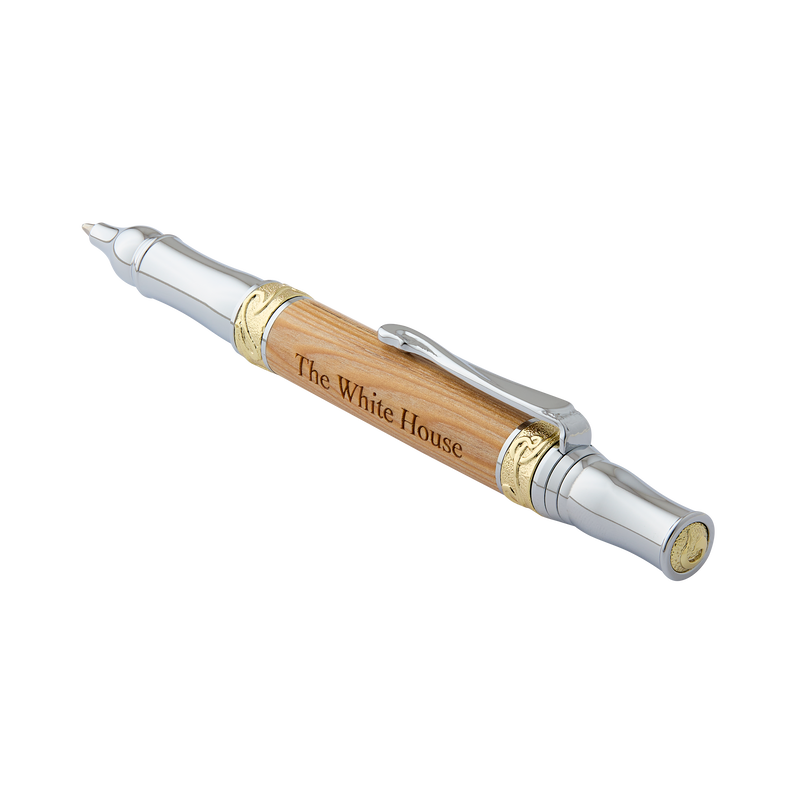In this close-up image set against a white background, a luxurious yet seemingly commercial pen lies diagonally with its writing tip positioned in the upper left corner. The pen's body is predominantly made of shiny, light gray metal, likely plastic or aluminum, giving it a somewhat cheap yet polished appearance. The middle section of the pen features a long, light tan, polished wood cylinder, prominently branded with "The White House" in darkened brown lettering. This wooden section is flanked by small, round golden bands embossed with intricate designs, adding a touch of ornate elegance. At the top of the pen, a silver clip is attached for securing it to a shirt pocket, enhancing its practical appeal. The pen is further adorned with a gold medallion at its top, completing its sophisticated yet tourist-oriented design.